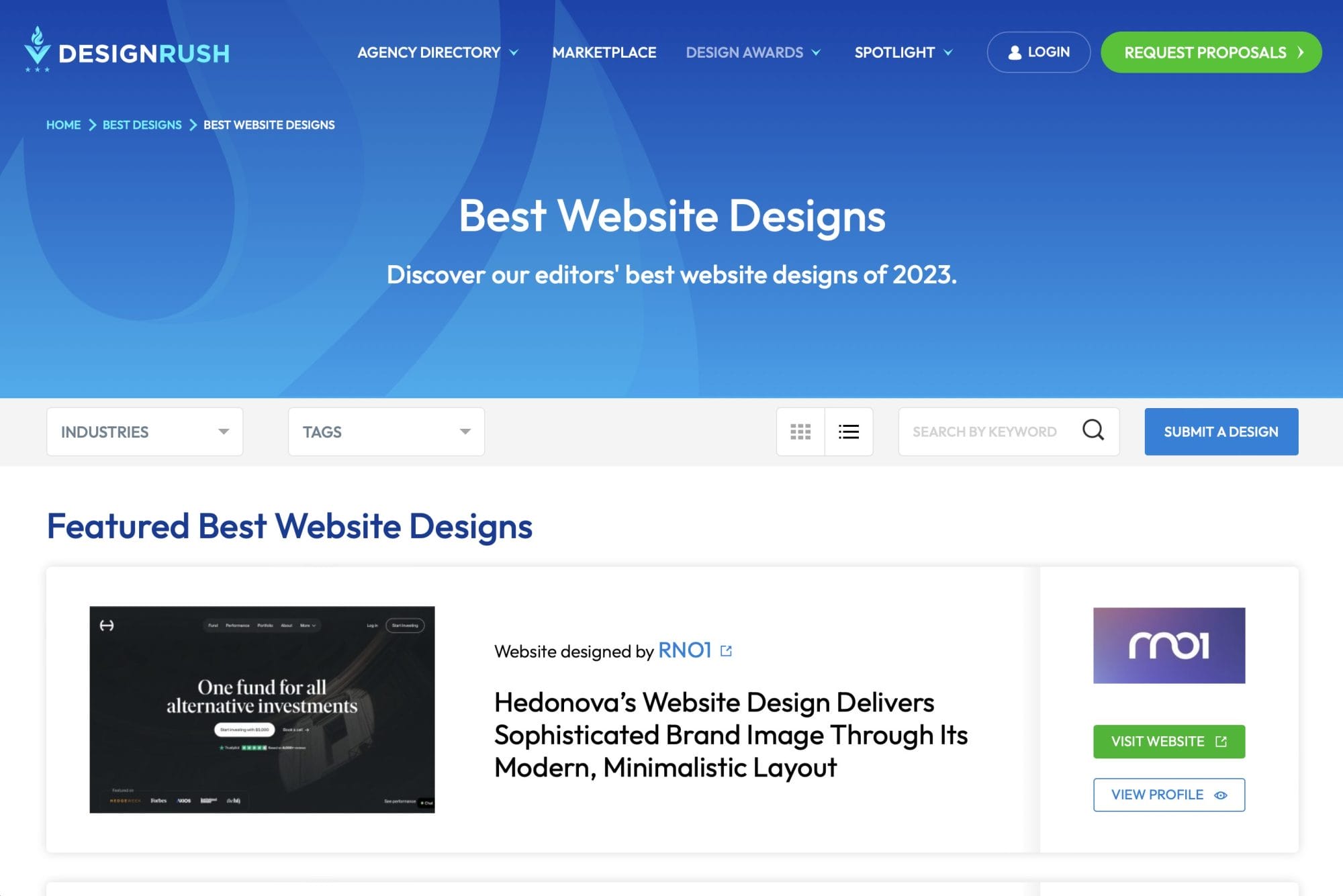The top portion of the image features a light blue banner. On the left side of the banner, there's a gradient design that transitions into a lighter blue. Bold, capitalized text states "DESIGN RUSH." To the right, a menu includes various options: "HC Directory," "Marketplace," "Design Award," "Spotlight," "Login," and "Request for Proposals."

Below the top banner is another navigation menu with options such as "Home," "Best Designs," and "Best Website Designs." Prominently displayed beneath is the title "Best Website Designs" in large white letters. Underneath this, smaller text reads, "Discover our Editors' Best Website Designs of 2023."

The background transitions into a white section containing two drop-down menus, labeled "Industries" and "Tags," respectively. Adjacent to these is a search bar with a magnifying glass icon, and a blue button marked "Submit a Design."

Further down, the section titled "Featured Best Website Designs" is presented in dark blue text. Below this heading is a video player, suggesting that you can watch a video. To the right of the video, text describes a specific design: "Hedonova's Website Design delivers sophisticated brand image through its modern minimalist layout."